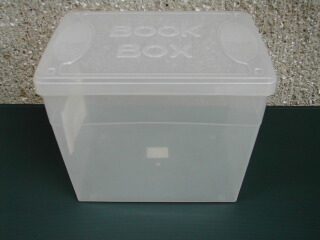In the image, a single object commands attention, positioned directly in the center against a textured background. The setting appears to be outdoors, perhaps against someone's house, indicated by the stone or pebble masonry wall in the background. The object is a plastic container with an opaque, glazed look, presenting a hint of translucency but not entirely clear. The container is labeled "book box" on the top, with no other visible markings. The photography angle is from above, allowing a view of both the top and one side of the container. It rests on a surface that could be painted pavement or a table or stand, with a dark hue that might be black, dark gray, or navy blue. The colors in the image are predominantly shades of gray, white, and a hint of greenish color, enhancing the detailed textures and solid surfaces in the scene.